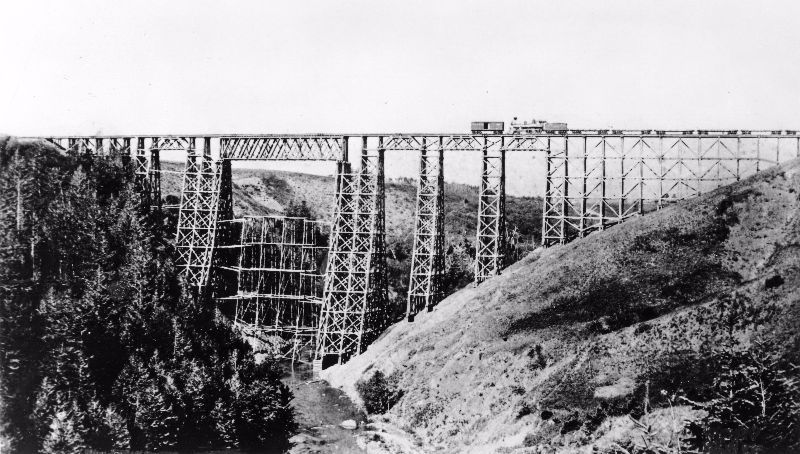This black and white photograph, likely taken around the late 1800s or early 1900s, captures a dramatic landscape in a landscape layout, with the horizontal dimension being longer than the vertical. The primary focus is a majestic wooden bridge, resembling the intricate lattice of the Eiffel Tower, spanning a wide and deep valley. The valley's floor is home to a winding river, framed by a dense forest of redwood and pine trees on the left side. On the right, the terrain ascends into a rocky hill.

High above the valley floor, the bridge is supported by a network of tall, vertical columns and smaller structures, creating an impressive engineering feat. On this bridge, a locomotive pulls a series of about five or six flat train cars and a box car, making its way across the valley from the left mountaintop to the right. The sky forms a distant backdrop to this timeless scene, highlighting the isolation and grandeur of the early railroad construction era.